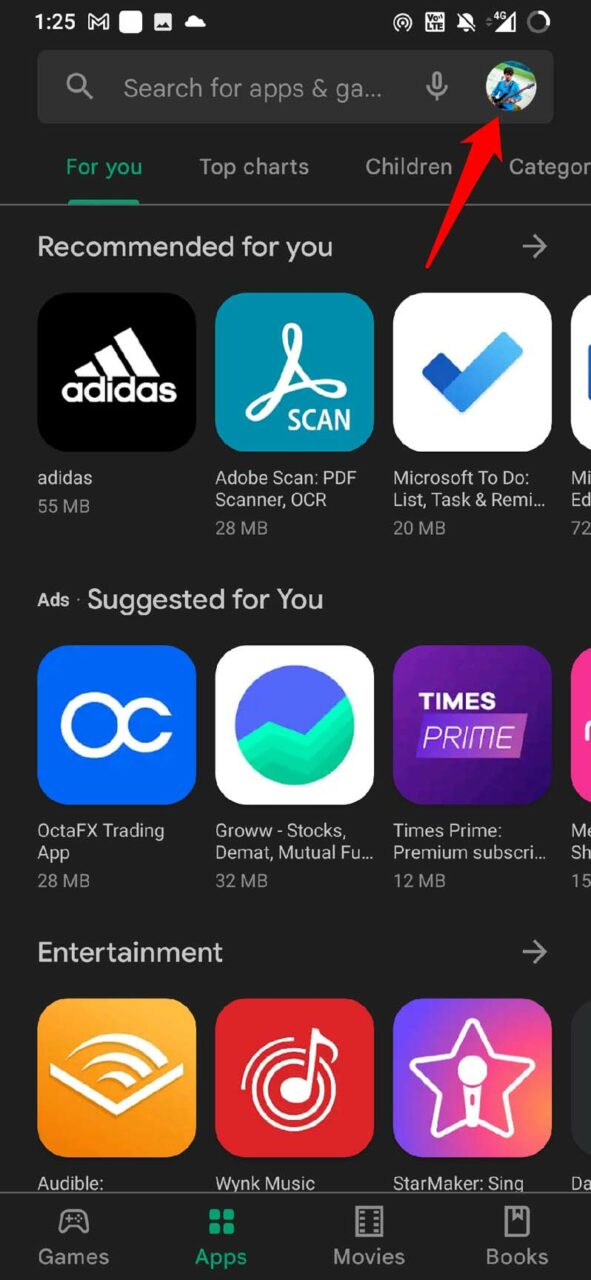This is a detailed screenshot from an iPhone showcasing the App Store interface. The background is predominantly black, which is typical of the dark mode setting. 

In the upper-left corner of the screen, various pieces of information about the phone are displayed in white font. The time reads 1:25 PM. Beneath the time, there is a notification icon for a new Gmail message. There are additional icons visible: a white square, a photo icon, and a cloud icon. 

On the right side of the top bar, the phone's signal strength icon is visible along with other unidentifiable icons due to their small size.

Beneath this top bar is a grey search field. On the left of the search bar, there is a small magnifying glass icon, indicating the search functionality. The grey font inside the search field instructs the user to "Search for apps and games...". Adjacent to this text on the right is a grey microphone icon, suggesting voice search capability. Further right, there is a profile picture of the user, which shows a man holding a guitar. This profile picture is highlighted by a photoshopped red arrow, indicating its significance.

Below the search field, the screen displays navigation tabs: 'For You', 'Top Charts', 'Children', and 'Categories', all in grey font. The 'For You' tab is selected, indicated by its underline.

In the main content area of the screen, several app recommendations are given. These include the Adidas app, Adobe Scan app, and Microsoft To-Do list app, tailored specifically for this user.

The meticulous arrangement and highlighted elements suggest a focus on personalized content and user engagement within the App Store interface.